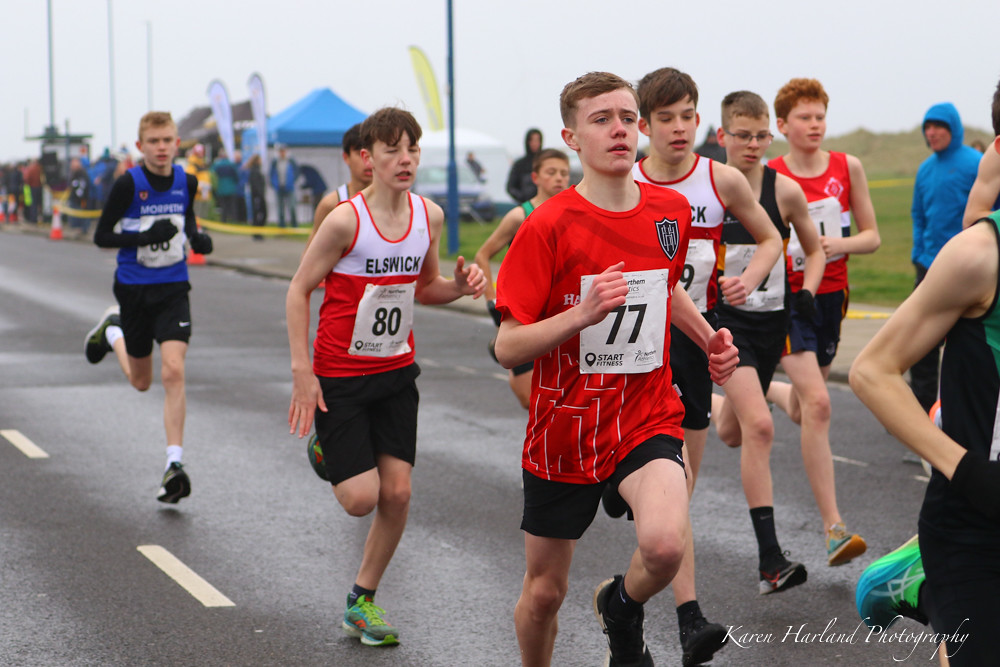This detailed photograph captures a group of about ten young boys, likely in their mid-teens, running a distance race, presumably a marathon or a cross-country event given their road setting. The chilly, overcast day suggests a cold and possibly rainy environment, as indicated by the wet asphalt road and the blue hooded parka worn by a spectator on the right side of the image. The boys are running down the middle of the road, which is devoid of any other traffic. 

The leading boy, prominently visible on the right edge of the frame, wears a red T-shirt, black running shorts, and black shoes, with a number "77" pinned to his chest. Trailing him closely, another runner dons a white and red tank top with the number "80." Most of the boys are in red or red and white attire, and all are wearing black shorts. The boy at the back is distinct in a long-sleeve blue and black outfit. 

Surrounding the race are blurred spectators and various tents and banners, with a yellow strip cordoning off the area where the audience stands. In the distance, green hills rise behind the chaotic collection of people and stands. Despite the dynamic activity, the runners maintain clear focus in the image, contrasting the slightly out-of-focus background. The lower right corner bears the watermark "Karen Harland Photography," suggesting the photographer's professionalism and attention to branding. Overall, the scene is set in a picturesque, likely British countryside, emphasizing the communal and competitive spirit of the event.